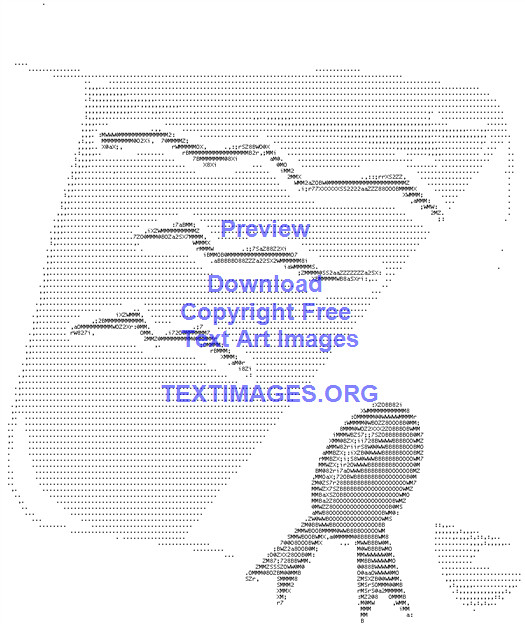The image appears to be a form of text art, crafted by arranging various symbols and characters to create visual impressions. Dominating the left side of the predominantly white image with gray dots is a representation of a mask-like outline, which intriguingly features three zigzag lines extending down the middle. This mask portion fills roughly 70% of the left side of the image. On the right side, there is a darker gray element resembling an egg, from which ribbons emanate at the bottom. Centrally located blue text reads, "Preview, download, copyright-free, text art images, textimages.org." This text breaks up the visual elements and provides a clear focal point for the viewers.